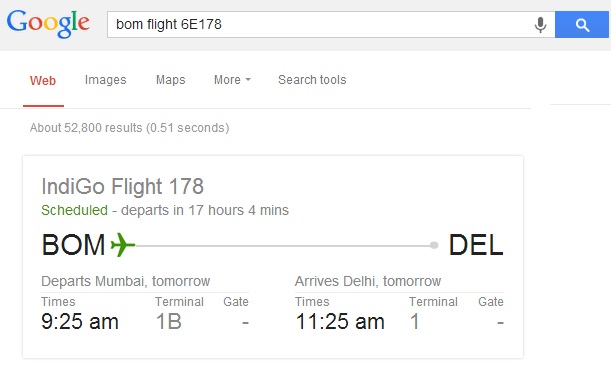In this Google search page screenshot for a flight schedule, the interface features Google's logo in a grey box at the top, accompanied by a search bar containing the query "BOM flight 6E17A" and icons for a microphone and a magnifying glass on either side of the bar. Below the Google header, the 'Web' option in red and underlined indicates the selected search category, with adjacent options for 'Images', 'Maps', 'More', and 'Search tools' also visible.

The search results indicate approximately 52,800 matches, with the first result presented in a highlighted box. This box displays information about Indigo Flight 178, scheduled to depart in 17 hours and 4 minutes. The flight details inside the box show "BOM" (Chhatrapati Shivaji Maharaj International Airport, Mumbai) on one side of an airplane icon followed by "DEL" (Indira Gandhi International Airport, Delhi) on the other side. Below this, it specifies the departure from Mumbai at 9:25 AM tomorrow, from Terminal 1B, Gate unspecified. The arrival in Delhi is noted to be at 11:25 AM tomorrow, arriving at Terminal 1.